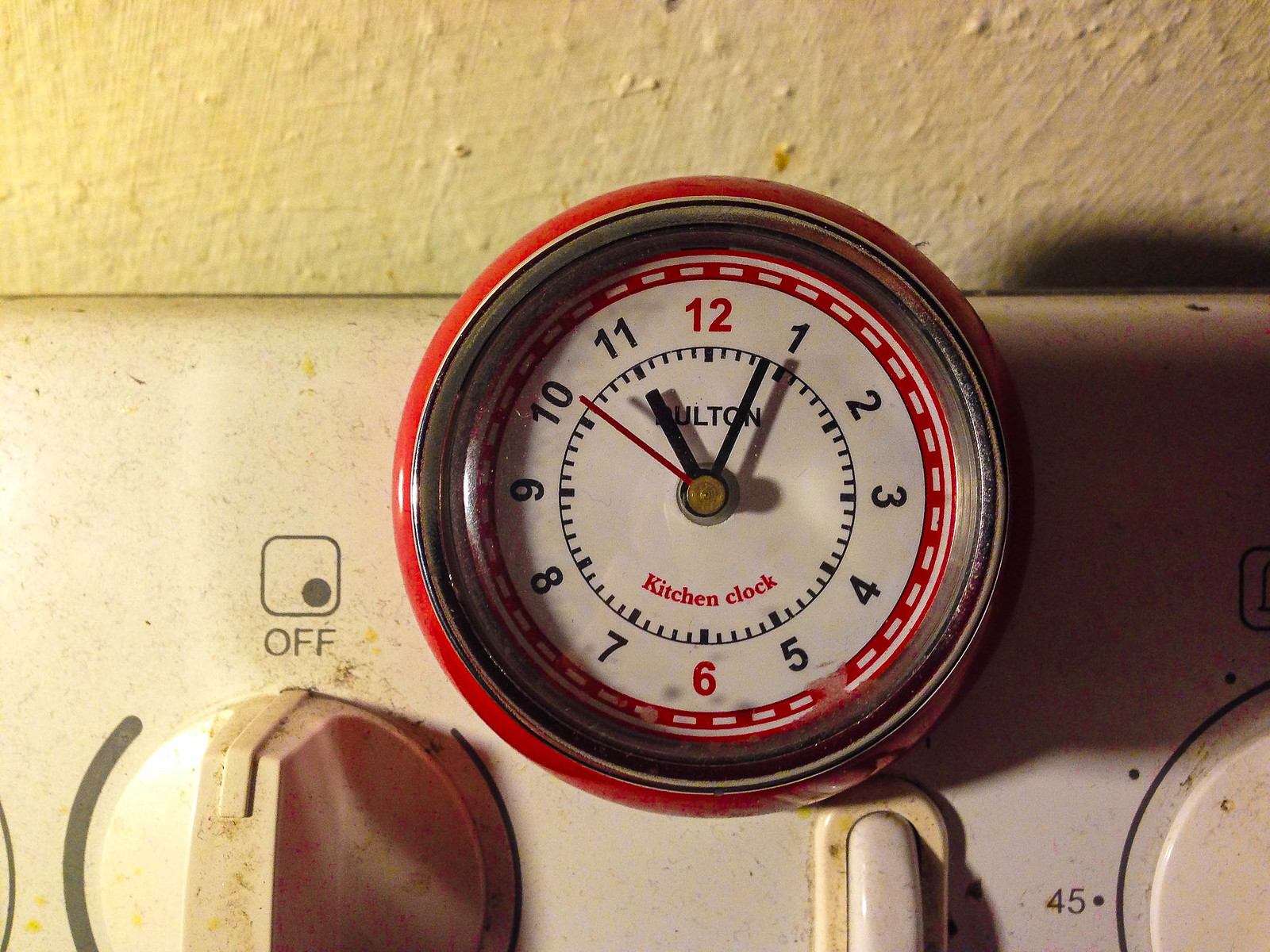In the center of the image, a circular clock stands out prominently. The clock features a double red border – a striking red outer edge and a slightly more subdued red inner circle. The face of the clock is white, providing a stark contrast to its frame. Unconventionally, the numbers are arranged in a counterclockwise direction. The number 12 and number 6 are highlighted in red, while the remaining numbers are in black. The clock has three hands: two are black, and the third is a vibrant red. At the bottom, the words "kitchen clock" are written in red, matching the color scheme of the borders and select numbers. The clock is mounted against a white wall, which is visible in the upper background, and it appears to be attached to a white machine below it.